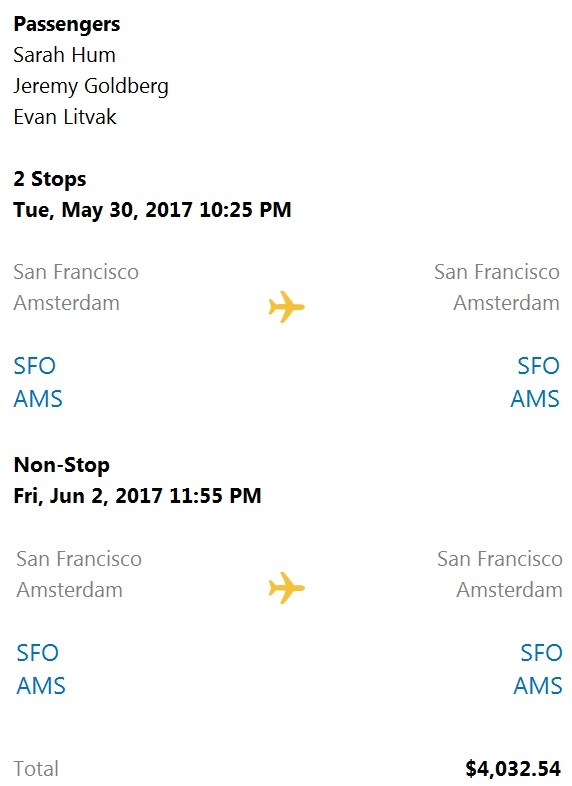Here is a cleaned-up and detailed caption for the image:

"This screenshot depicts an itinerary page characterized by a predominantly white background. At the top left corner, 'Passengers' is prominently displayed in bold black text, followed by a list of names: Sarah Hum, Jeremy Goldberg, and Evan Litvack, each on a separate line. Directly underneath this, the text reads 'Two stops,' accompanied by the date 'Tuesday, May 30, 2017,' and the time '10:25 PM.' Below this information, the route 'San Francisco to Amsterdam' is shown in gray text flanked by a yellow plane icon in the middle. To the right, the route 'San Francisco to Amsterdam' is repeated. The airport codes 'SFO' and 'AMS' are shown in blue text on both ends of the route. Further down, details for a nonstop flight on 'Friday, June 2, 2017,' at '11:55 PM' are provided, indicating travel between the same two locations. At the bottom of the page, the total cost is listed as $4,032.54."